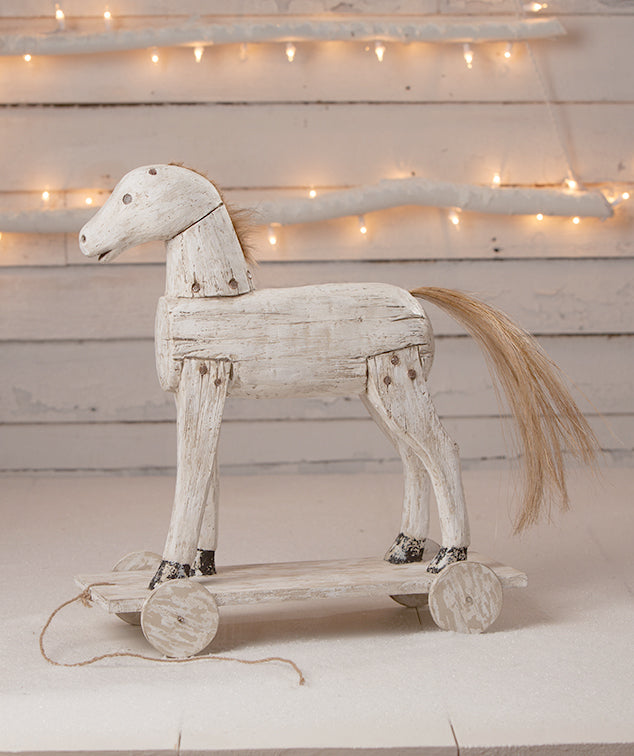The image depicts a vintage wooden pull toy in the shape of a horse, set against a distressed, whitewashed wooden backdrop with two rows of fairy lights. The horse, standing on a whitewashed platform with wooden wheels, showcases signs of wear and age—the smooth, worn wood, chipped white paint, and visible nailed or screwed joints bring out its weathered charm. The horse's mane, although full and long in the back, appears short and somewhat sparse in the front, suggesting some hair has been lost or cut over time. Its black hooves, likely once painted, exhibit a rustic appearance due to significant paint chipping. A hemp string is attached to the front, indicating its intended use as a pull toy for children. The floor beneath mimics the texture of snow, contrasting with the neutral tones of white, tan, and grey in the scene. The overall placement and intricate details—like the missing ear and the exposed cut portion of the log body—highlight the toy's antique allure.